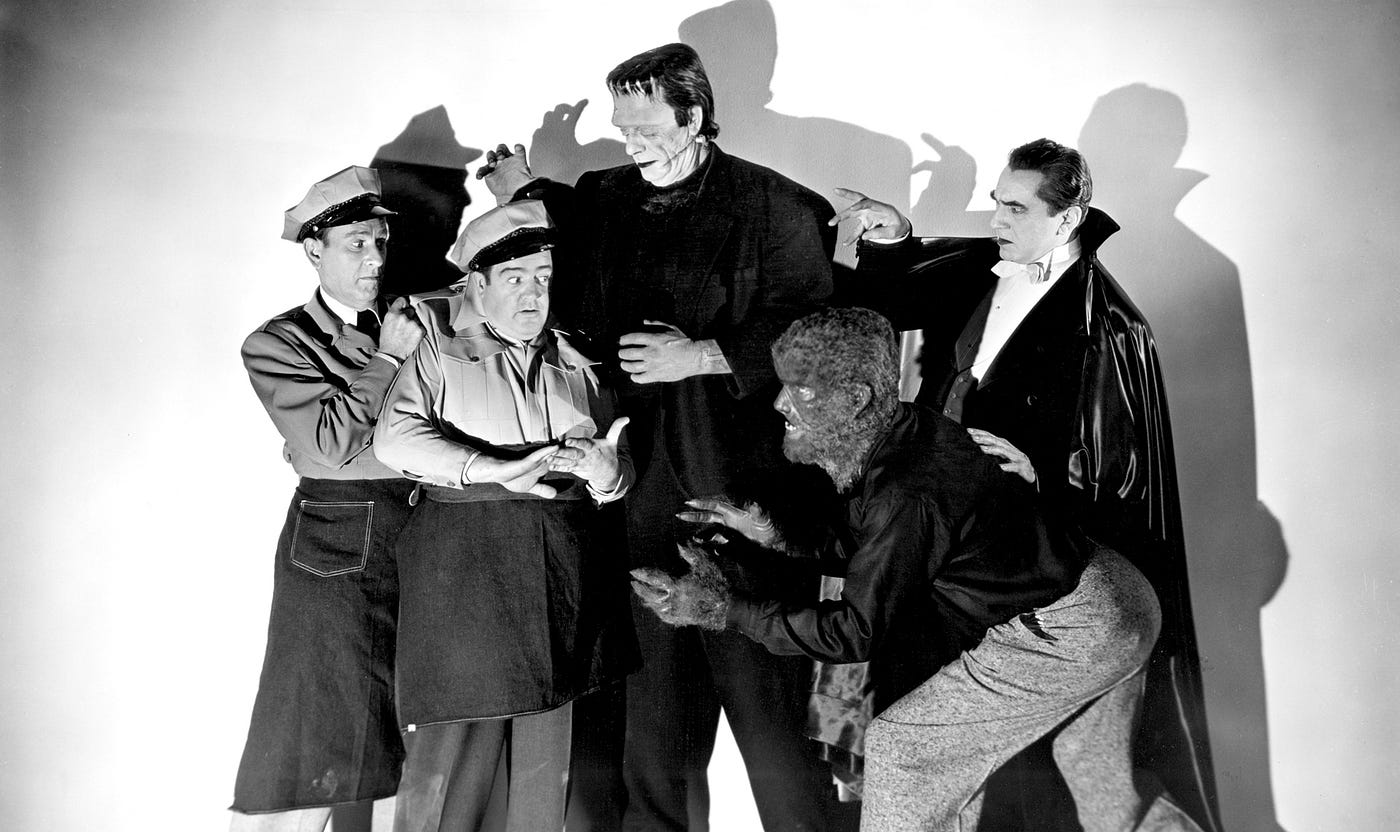The vintage black and white photograph showcases actors dressed in classic horror film costumes. Central to the image is Frankenstein's monster, towering over the scene with an imposing presence. On the right, a figure dressed as a vampire, likely Dracula, is clad in a long, dark cape and is positioned with a menacing stance, his right hand poised as if ready to attack. Crouched in front and to the right of him is a werewolf, complete with a furry mask and equally hairy hands, seemingly in the midst of a sinister interaction. On the left side of the photo, the comedic duo Abbott and Costello, recognizable by their caps and work uniforms, appear frightened as they confront these monstrous figures. The stark shadows in the white background enhance the eerie atmosphere, contributing to the overall menacing mood of this high-resolution depiction.